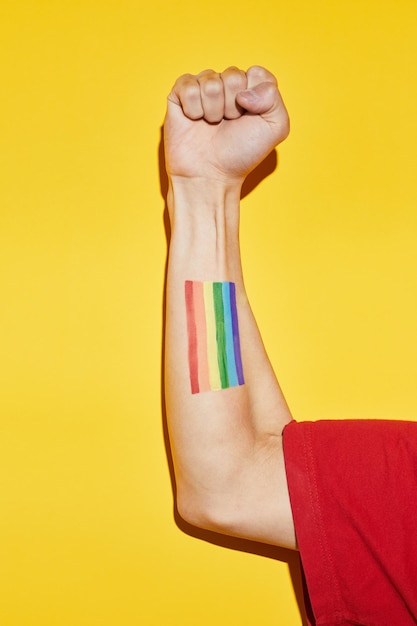In this vertically oriented, close-up photograph, a right arm is prominently featured against a bright yellow background, casting a distinct shadow. The arm, belonging to a light-skinned individual of indeterminate gender, is raised at a 90-degree angle with a clenched fist pointing upward. The person is wearing a short-sleeved red shirt, revealing just the bicep and forearm. On the forearm, there's a vividly painted or marked rainbow flag-like rectangle with stripes running vertically, displaying colors from top to bottom: red, orange, yellow, green, blue, and purple. The image captures a striking contrast between the bright yellow wall, the red shirt, and the colorful rainbow artwork, suggesting themes of pride or solidarity.